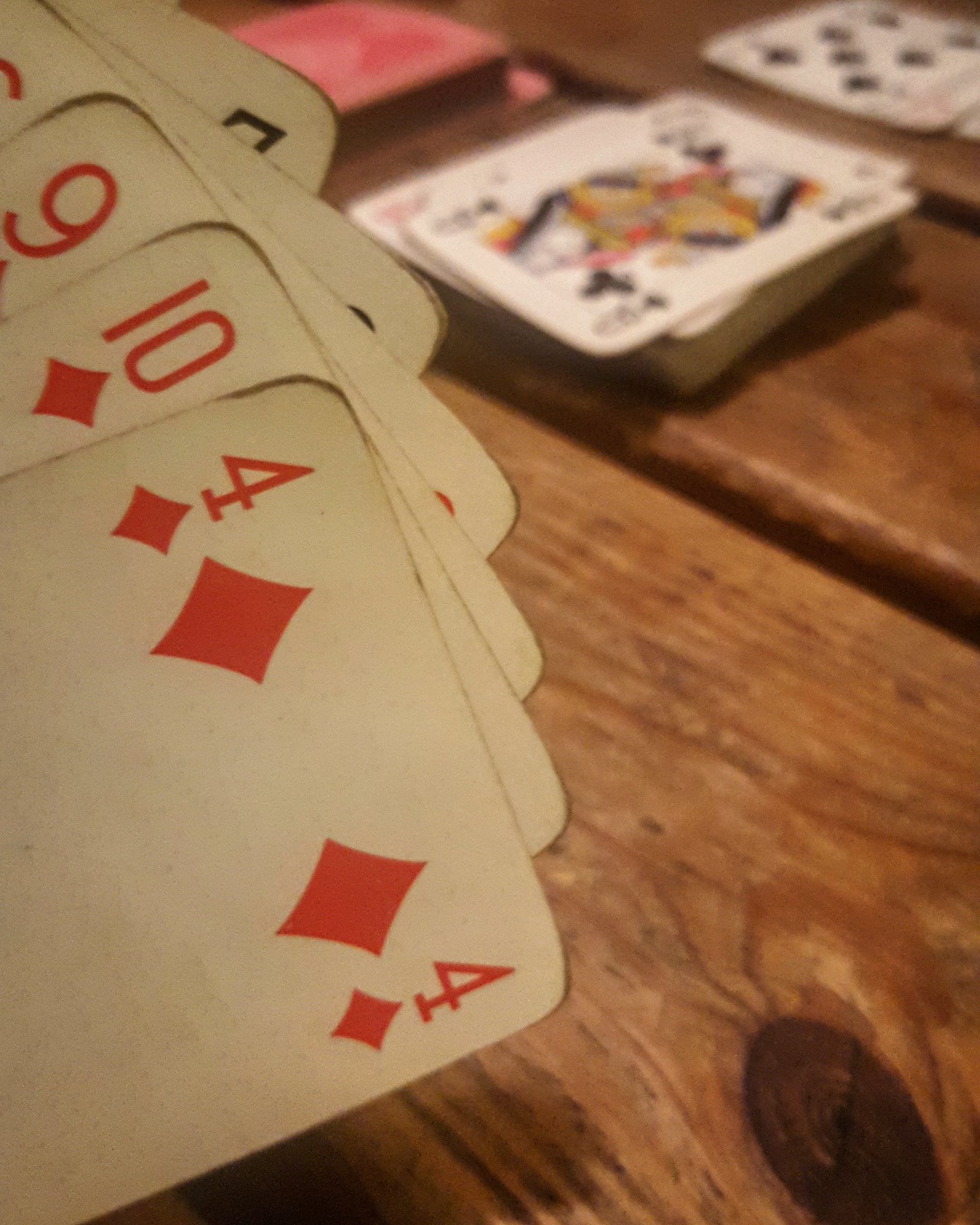In the image, a hand is holding a set of playing cards over a rustic picnic table, revealing six to seven cards only partially visible at the tops. The cards are strategically positioned so that the opponent across the table cannot see them. The visible cards include the four of diamonds, ten of diamonds, and nine of diamonds, accompanied by a six of an indistinct red suit, and two black cards, including a seven whose suit is not visible. On the table below, an organized deck displays face-up cards, and another deck or card box lies face down. The opponent's cards are laid out face-up on the table, indicating an ongoing game. The scene portrays a casual yet intensely strategic moment in a card game, set against the backdrop of a charming outdoor setting.